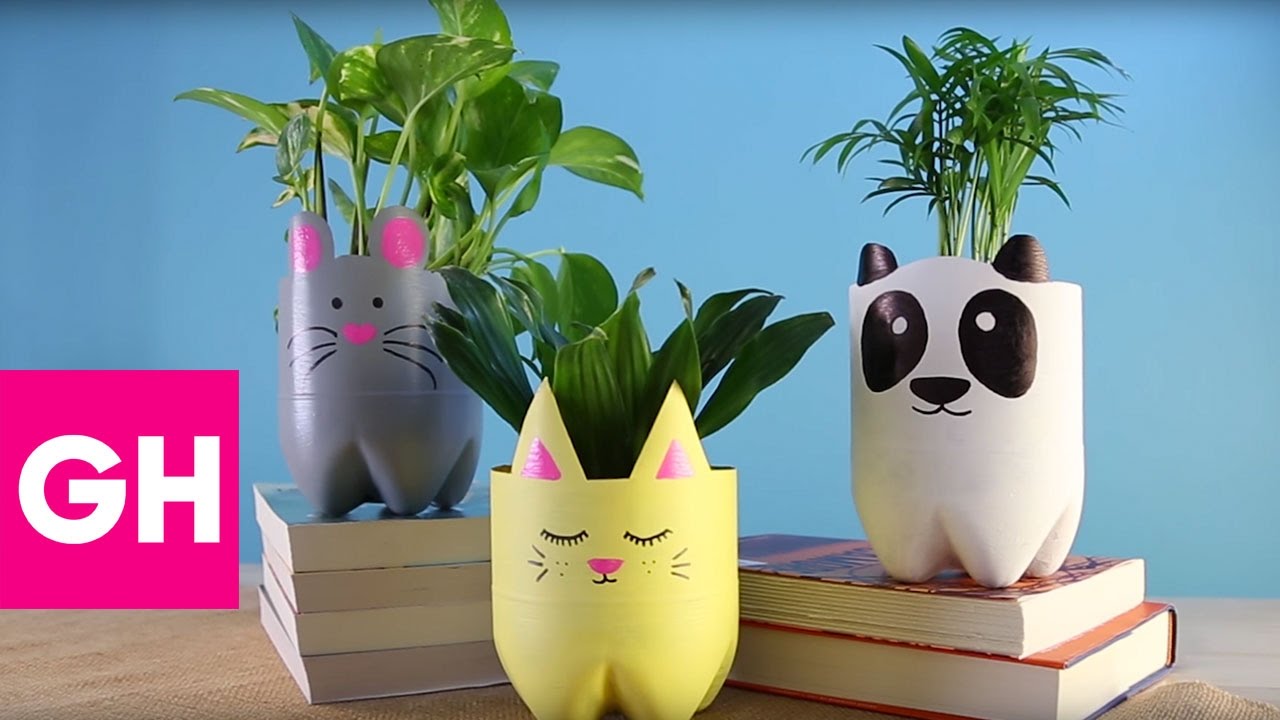In this vibrant image, a blue wall serves as the backdrop for a creative display of handcrafted flower pots made from repurposed two-liter bottles. Arranged on a table or bookshelf layered with various grey to light brown fabrics, the scene is adorned with a variety of books. On the right, two books are stacked—one hardcover and the other a paperback, while on the left, there are four additional paperbacks. Front and center is a yellow cat flower pot, its eyes closed, adorned with a pink nose, pink ears, and whiskers. A lush, leafy green plant sprouts from the top. To the right, a panda-themed pot painted in black and white holds another vibrant plant, and to the left, a whimsically styled gray mouse pot features a pink nose, beady eyes, and pink ears, also with a flourishing plant. A magenta square with the white capital letters "GH" is prominently visible in the lower left corner of the image, adding a pop of color and a hint of branding.